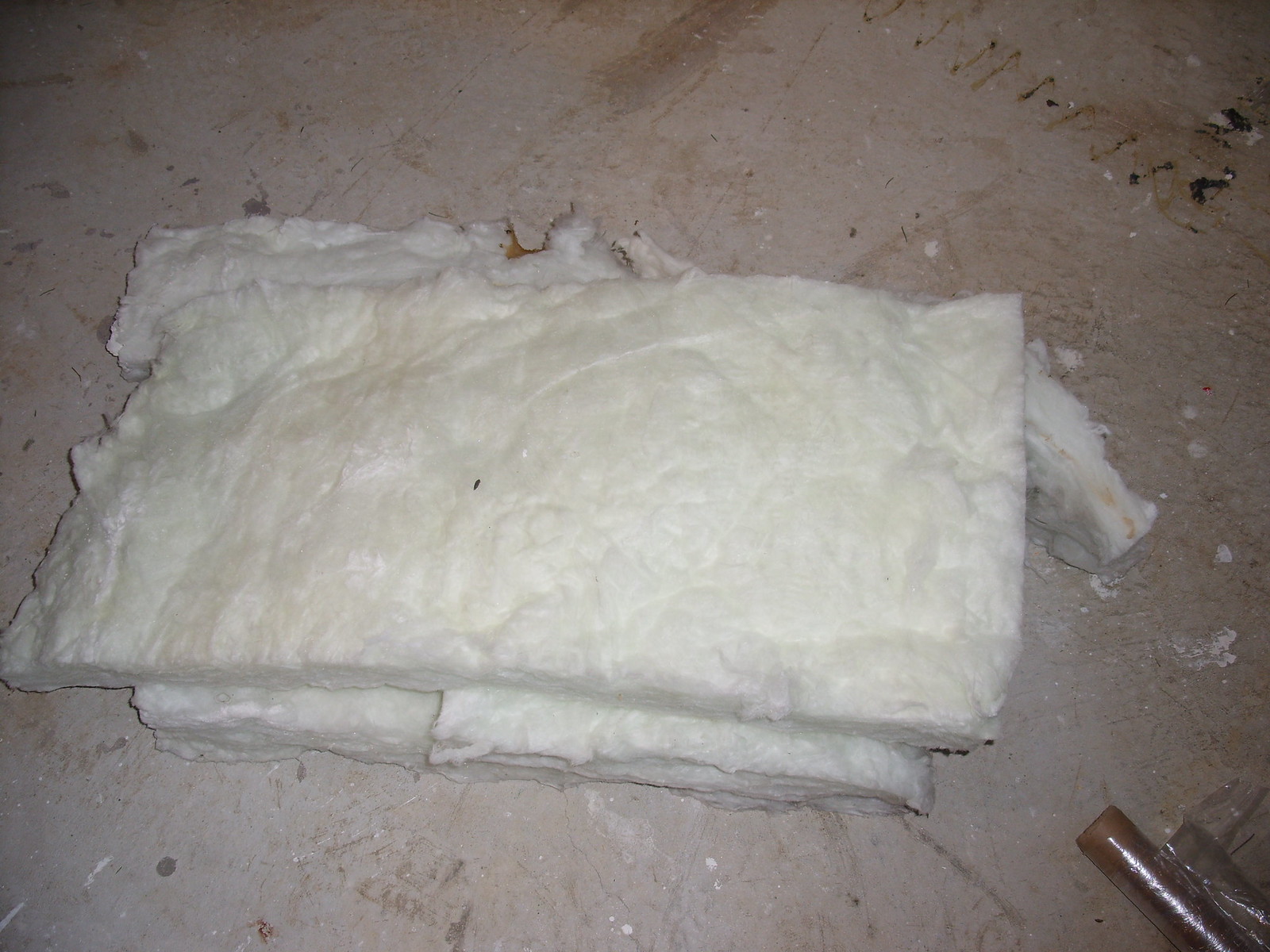The photograph captures a close-up view of old, used insulation material lying on a dirty, tan-colored cement floor, likely at a construction or renovation site. This insulation appears to be a thick, wooly cotton-like pad, folded over and stained, suggesting it's been pulled from its original placement, possibly during renovation. Surrounding the main chunk of insulation are smaller tufts and pieces scattered across the floor. In the lower right corner, rolls of plastic wrap can be seen. The insulation itself is situated in a rectangle shape, perhaps indicating there are two sections stacked together, and there's even a fly visible on one part of it, emphasizing its age and disarray.